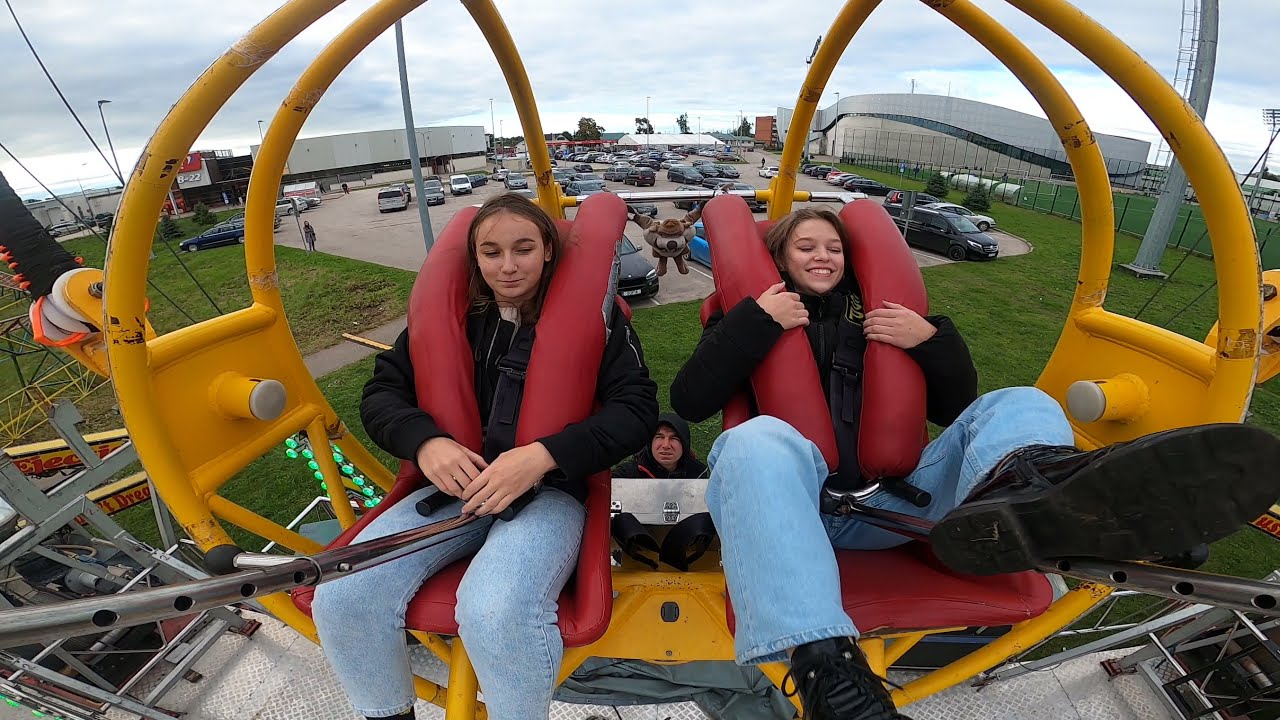In this vibrant daytime scene at an amusement park, two girls are the focal point, seated in padded red seats and secured by safety harnesses on a thrilling bungee ride. The ride's prominent yellow metal frame surrounds them, complemented by the silver rods and rails of the structure. Both girls sport black jackets and blue jeans, their expressions a mix of excitement and nervous anticipation. Positioned centrally, one girl sits slightly to the left while the other is to the right. Between them stands a man, possibly a ride operator, dressed in a hoodie.

The background features several key elements that add context to the image. A parking lot filled with cars of various colors—blues, blacks, and whites—expands behind them, interspersed with patches of green grass. Two large buildings occupy the corners of the frame, with one in the top left and another in the top right, both contributing to the bustling ambiance of the park. Above, the sky is a blend of blue with white clouds, adding a serene contrast to the energetic scene below. The overall image captures a moment of anticipation and joy, set against the dynamic backdrop of an adventure-filled amusement park.